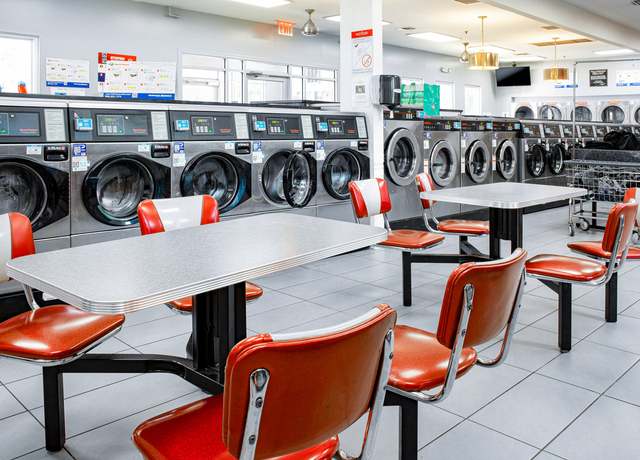The photograph captures the interior of a laundromat with notable precision and detail. The floor is covered with grey tiles, complementing the room's overall grayscale aesthetic. Centrally placed are two silver-lined tables, each supported by black stands and legs. These tables are flanked by orange-backed and seated chairs, attached to the tables' black legs, featuring a distinctive silver stripe down their backs.

In the background, there is a row of washing machines and dryers, extending from left to right in a slight angle towards the right and back. The machines are organized into two groups based on the color of their circular door frames: some have black circles surrounding the glass doors, while others feature silver circles. Notably, there are five silver washing machines prominently visible, with glossy grey fronts and immaculate glass windows in their doors. Above each machine, a black rectangle is equipped with various white buttons and blue screens.

Behind the row of machines, a grey wall is inset with numerous windows framed in white. A teal blue box is conspicuously placed atop one of the centrally located machines with a silver circle. The ceiling, painted white, is adorned with various light fixtures, including two gold-colored chandeliers hanging on the right side. The laundromat's design is both functional and visually cohesive, providing a clean and modern atmosphere for its patrons.